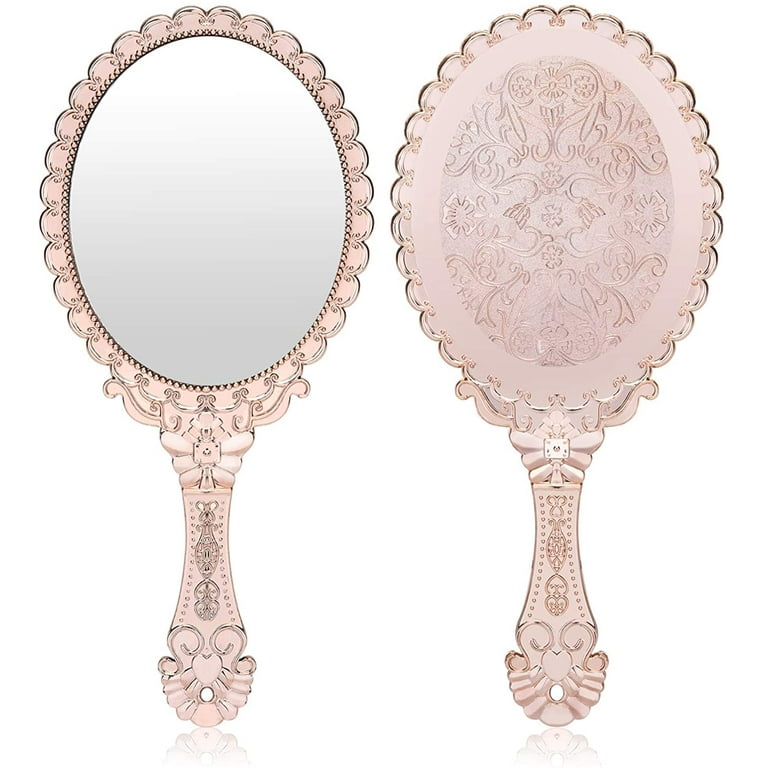This image features a side-by-side view of the front and back of a single ornate handheld mirror, predominantly pink in color, often referred to as rose gold. The mirror boasts a semi-circular lace pattern around its edges, adorned with small, intricate bows and floral designs. The handle, long and carved with a detailed scroll pattern, includes a decorative centerpiece connecting to the mirror. The backside mirrors the elaborate designs of the front, continuing the floral and bow motifs. Notably, the handle has a small hole at the bottom, allowing for it to be hung. This exquisitely designed mirror harkens back to the elaborate aesthetics of Victorian times.